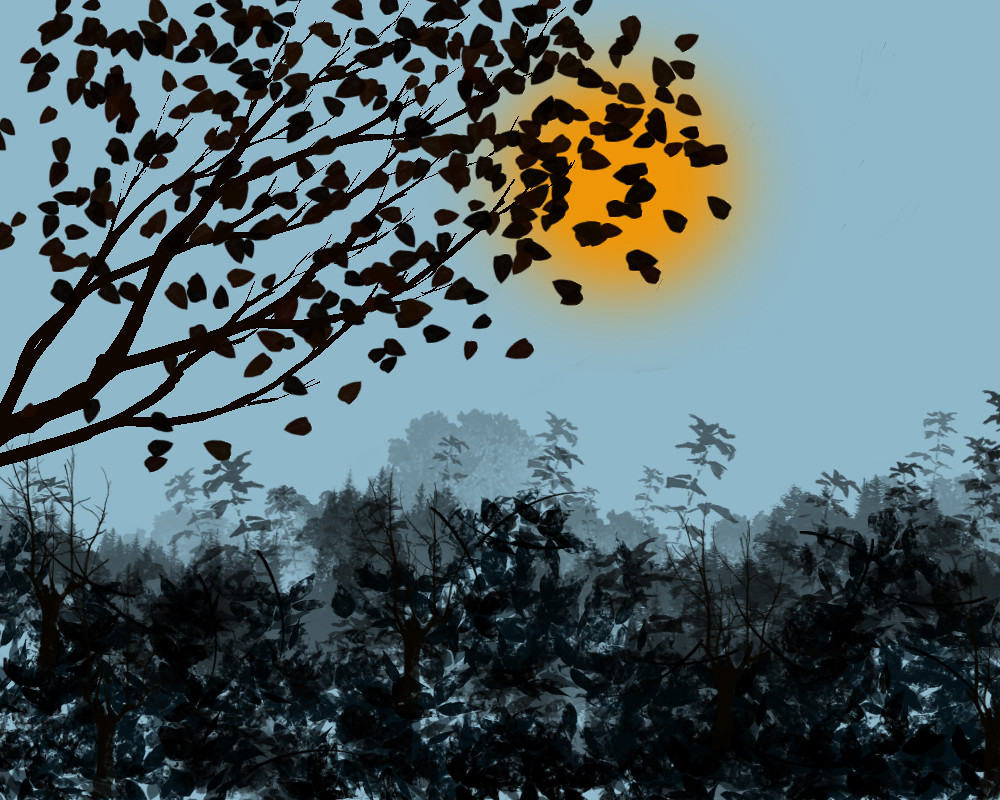This photograph captures the serene beauty of either a sunset or a sunrise. Dominating the background is a radiant, golden sun that casts a warm glow across the scene. The sky surrounding the sun transitions into muted shades of blue, contrasting sharply with the silhouetted foliage in the foreground. 

On the left side of the image, a tall tree, with leaves appearing to fall, stretches upwards, creating a striking silhouette against the sky. Below it, shorter trees or bushes add layers of depth to the composition, their forms becoming less distinct and more ethereal as they recede into the distance.

The foreground features dark, shadowed leaves, while the foliage further back fades into lighter shades of gray, beautifully illustrating the perspective and depth of the scene. In the distance, a larger tree stands out with a light gray, almost bluish, translucent appearance, adding to the mystical quality of the landscape.

Overall, the photograph is a harmonious blend of vibrant yellows and a subdued blue-gray palette, creating a tranquil and evocative depiction of nature at either dawn or dusk.